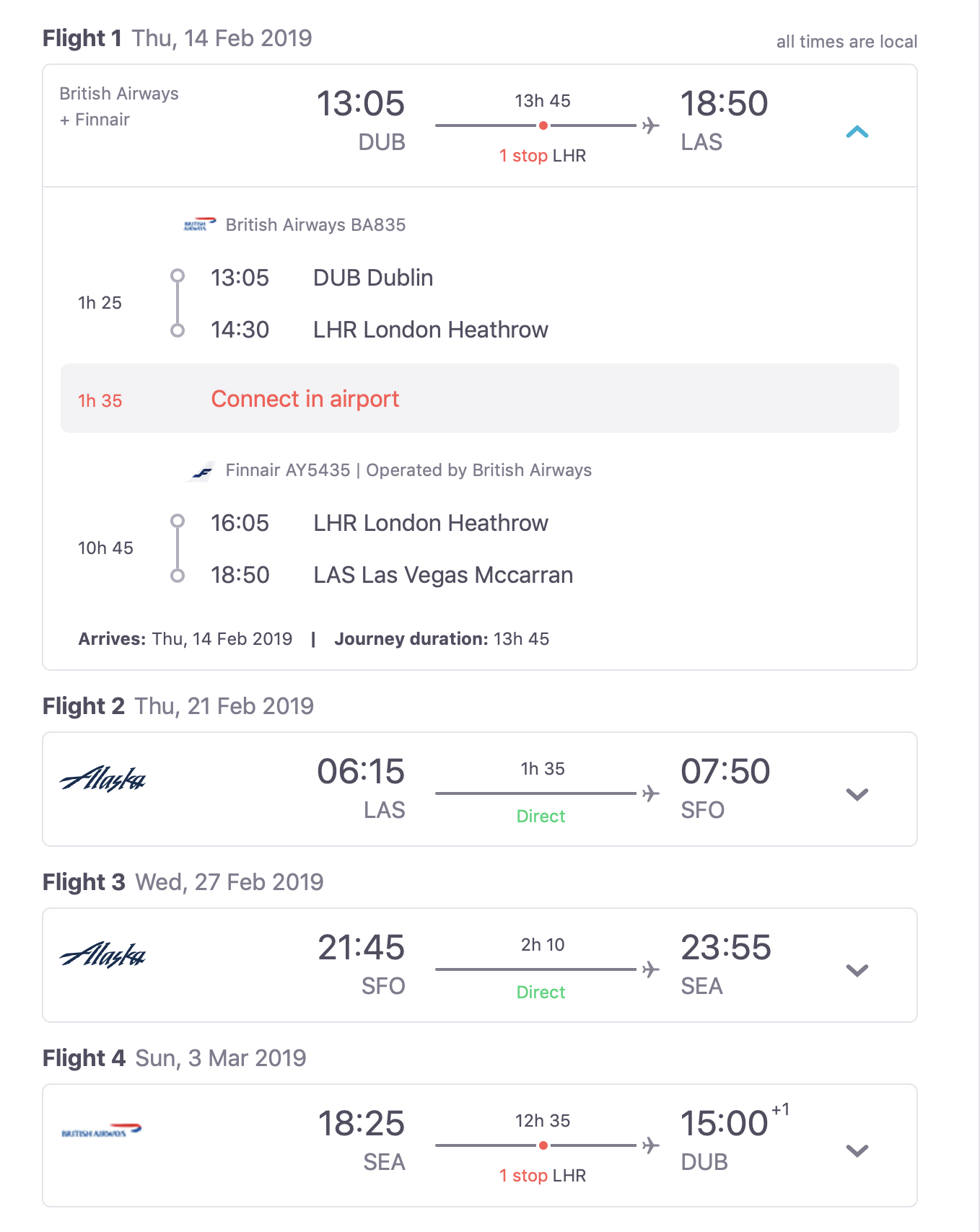**Detailed Caption:**

This color image appears to be a screenshot from a travel booking website, detailing flight information for a multi-leg journey. 

- **Flight 1:** 
  - Departing on Thursday, 14th February 2019 at 13:05 from Dublin (DUB)
  - Arriving at 18:50 in Las Vegas (LAS) after a total journey time of 13 hours and 45 minutes.
  - The first leg details British Airways flight BA35:
    - Departing Dublin at 13:05
    - Arriving at London Heathrow (LHR) at 14:30.
  - The second leg continues with British Airways (operating as AY5435):
    - Departing London Heathrow at 16:05
    - Arriving in Las Vegas at 18:50.
  - There is a total journey time of 13 hours and 45 minutes, considering a lengthy layover at London Heathrow. 

- **Flight 2:**
  - Departing Las Vegas (LAS) at 06:15
  - Arriving in San Francisco (SFO) at 07:50.

- **Flight 3:**
  - On Wednesday, 27th February 2019:
    - Departing San Francisco (SFO) at 21:45
    - Arriving in an unspecified destination labeled as "SCA" at 23:55. Note: "SCA" appears to be a typo or an unclear airport code.

- **Flight 4:** 
  - On the return journey, likely with British Airways:
    - Departing "SCA" at 18:25
    - Arriving back in Dublin after a 12 hours and 35 minutes flight at 15:00 the following day.

This image provides a comprehensive look at the detailed flight itinerary involving multiple stops and connecting flights, spanning from Dublin to Las Vegas, and includes additional travel onward from Las Vegas to San Francisco and beyond. The return journey is noted to be particularly lengthy and indirect.